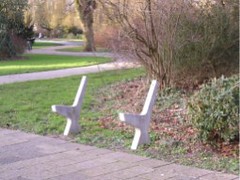A photograph captures an outdoor park scene bathed in sunlight, indicating a bright day possibly during fall or winter due to the presence of leafless trees and some brown leaves on the ground. Central to the image is a park bench frame sitting on a vibrant green grassy patch to the right of a winding, tiled sidewalk that cuts diagonally across the scene from the bottom right, zigzagging through the park and disappearing into the background. This bench frame consists only of two white cement posts where the wooden slats for sitting and backrest are missing. A large brown bush and a smaller green bush are positioned to the right and above the bench frame. The background reveals a mixture of massive bushes and trees stretching out to the upper left corner, where faint images of other benches are barely visible. The park has an overall open and peaceful ambiance, with the crispness of the season hinted at by the leafless trees and the clarity of the paths weaving among the greenery.